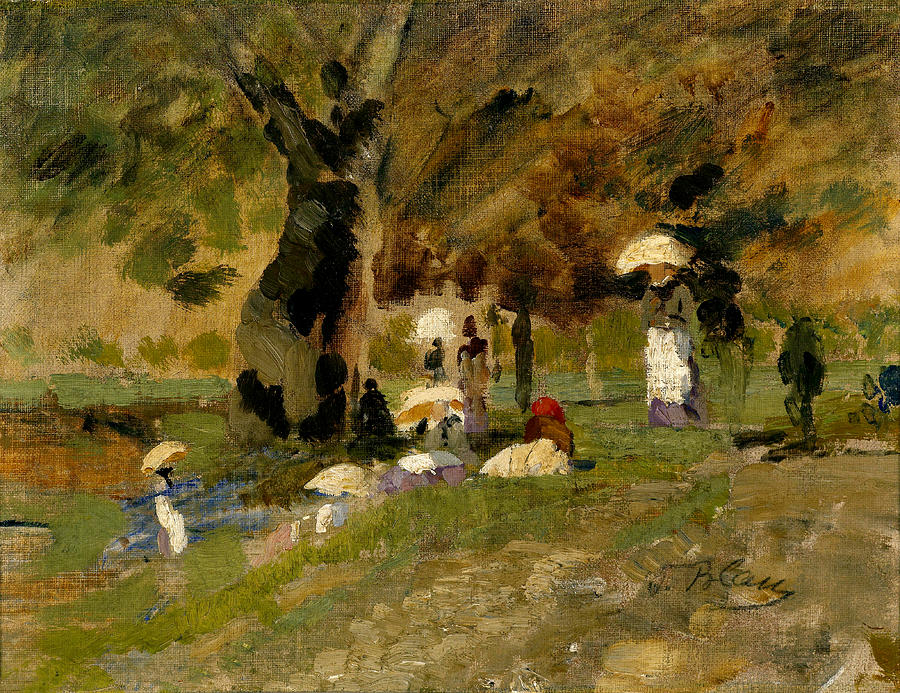This impressionistic oil painting depicts a serene outdoor scene, likely a park, bathed in olive, brown, green, and cream hues. The focal point is a large, bold-trunked tree positioned toward the left-center of the canvas, with its dark brown and black trunk and branches extending across the top of the composition, creating a leafy canopy in muted green tones. Beneath the tree, several women are picnicking; some sit on the ground in the foreground, adorned in long dresses and elaborate hats, and holding parasols that are more clearly defined than their figures, adding pops of yellow and white. One prominent figure to the left stands out in a purple dress with a brown long-sleeved top, a white apron, and a large yellowish parasol. The background features blurred green and cream hues, adding to the overall impressionistic style, with figures rendered in indistinct, brush-stroke details, giving a harmonious, fluid sense to the scene. The canvas's texture is visible through the brush strokes, further enhancing the painting's evocative quality. In the bottom right corner, the signature "J. Poole" can be discerned, though it is somewhat hard to read.